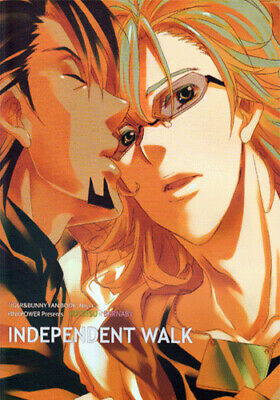The image is an abstract drawing of a man and a woman who appear to be a couple. The man, positioned on the left, has long black hair, a punk rock look, and a goatee. He is Caucasian with light yellowish skin, a pointy nose, a well-defined jawline, and is wearing a black shirt. The woman, taking up most of the right side, has lighter beige skin, striking red-orange hair, and wears angular beige glasses and a green necklace. Both characters have prominent features, with the woman's detailed more intensely. The drawing is predominantly in colors like black, red, orange, white, and green. The image features the text "INDEPENDENT WALK" in all capital letters at the bottom.